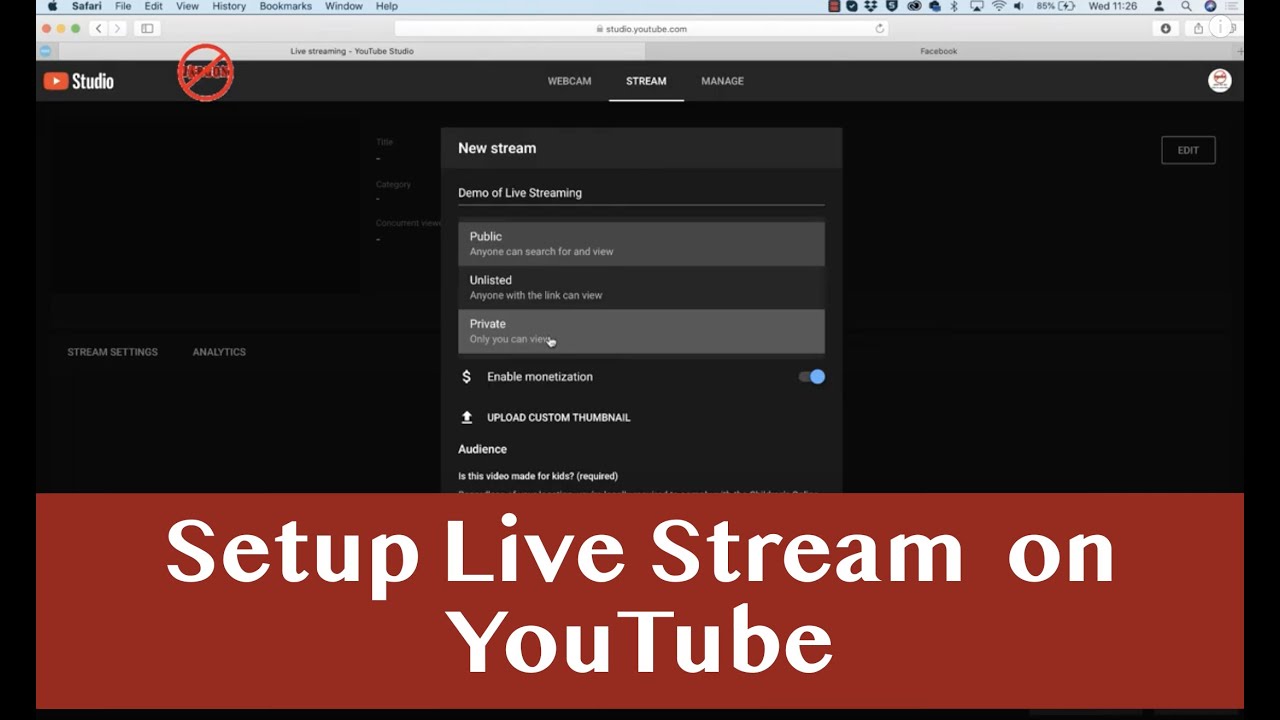**Detailed Caption:**

The image is a horizontal screenshot of a webpage displayed in the Safari browser. Centrally, a pop-up box is prominently visible against a jet black background. Above this box, a large red horizontal banner with bold white text reads, "Set Up Live Stream on YouTube." 

The Safari browser's heading bar at the top presents standard headings: File, Edit, View, History, Bookmarks, Window, and Help. To the bar's right, several icons are visible alongside the battery indicator and the current time. Directly below, a light gray address bar shows the URL studio.youtube.com.

To the right of the text "studio" within the address bar, there is a circular red icon with a line through it, with some text beside it. Below the address bar on the left, the YouTube icon is visible just above a gray scroll bar.

The pop-up box's main heading reads "New Stream, Demo of Live Streaming," with subsequent sections detailing the streaming options. The stream category has three subheadings: Webcam, Stream, and Manage, with "Stream" being underlined to indicate the current selection. 

The options within the pop-up are organized into categories, indicating the stream’s visibility status as Public and Private. Other options include "Unlisted," "Enable Monetization" (which is enabled), and an option to "Upload Custom Thumbnail."

The entire setup within the browser window is framed by a thin blue border, adding a subtle highlight to the interface elements.